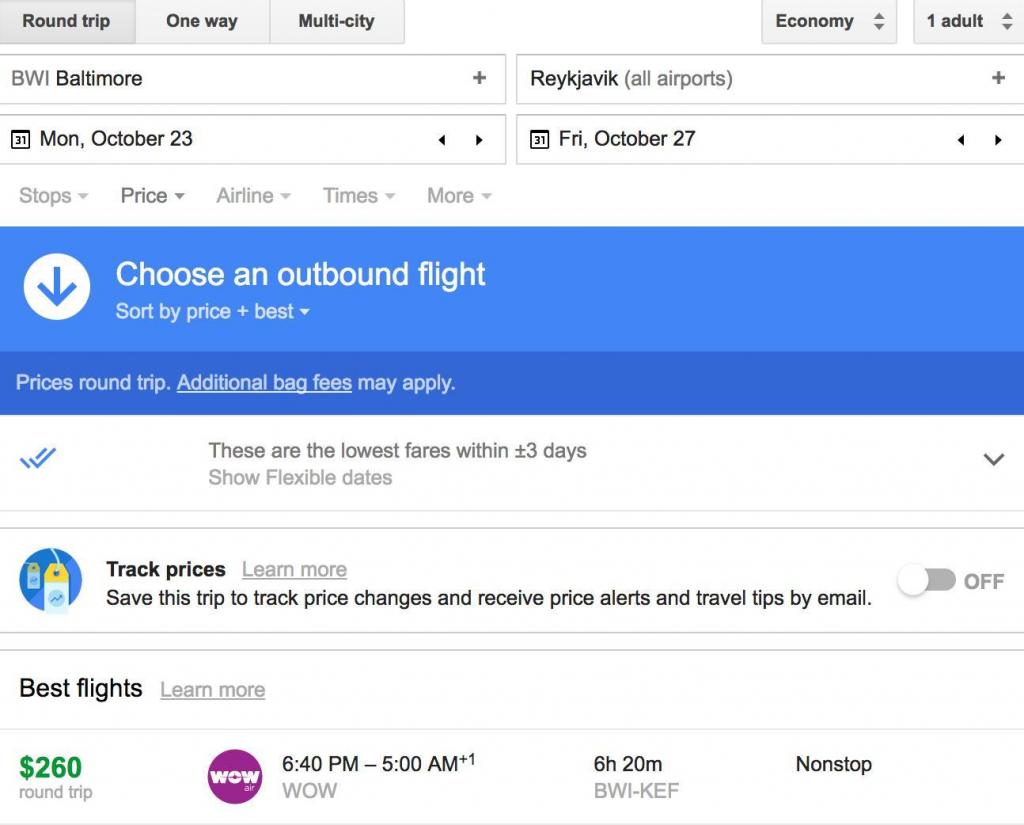The image displays a website interface for booking airplane seats. The top section features three tabs labeled "Round Trip," "One-Way," and "Multi-City," corresponding to different travel itineraries. Below these tabs are a couple of drop-down menus; one currently set to "Economy," with options likely including "Business" and "First Class," and another indicating "One Adult."

The travel details specify a journey from Baltimore (BWI) to Reykjavik, departing on Monday, October 23rd, and returning on Friday, October 27th. These details are selected via drop-down menus or fill-in fields for customizing the search.

Below the search criteria, there is a results section framed by a blue box with a downward arrow. It features an admonition to "Choose an outbound flight" and offers sorting options by price or other criteria. A note clarifies that prices are for round trips and may include additional baggage fees. There’s also a prompt with a double check mark stating, "These are the lowest fares within plus or minus three days," along with an option to "Show flexible dates."

An icon resembling a price tag introduces the "Track Prices" feature, which allows users to save the trip and receive price alerts and travel tips via email. This feature is currently turned off.

Finally, the "Best Flights" section lists one available flight, which appears to be partially clipped. The displayed flight costs $260 round trip, departing at 8:40 PM and arriving at 5:00 AM, with a total duration of 6 hours and 20 minutes for a nonstop, direct flight.